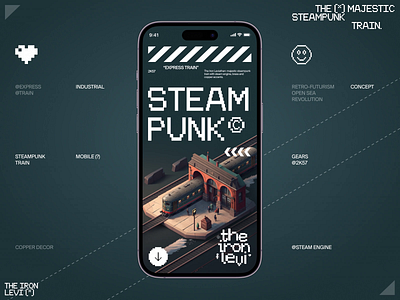This detailed illustration portrays a smartphone app advertisement set against a dark greenish-gray background. Dominating the center is the digital rendering of a phone, surrounded by small pixelated icons including a white heart, a smiley face, and a pixelated heart, symbolizing various categories like industrial concept.

At the top left corner of the background, white text reads "The Majestic Steampunk Train." Adjacent to that, inside the phone rendering, is the time "9:41" along with traditional smartphone symbols - a signal bar, a wireless symbol, and a battery indicator, followed by a series of white slanted lines and a swipe icon.

The centerpiece inside the phone screen features the word "Steampunk" in a pixel font, followed by a © symbol and the text "The Iron Lever," although parts are slightly obscured. Below this, a visually intriguing scene unfolds: a small train station with arches in red, through which a train traverses. The train tracks interestingly continue beyond the train station, transforming into a dotted line that integrates into the overall design.

The illustration underscores the nostalgic and mechanical aesthetics of steampunk, merging digital and vintage elements to create a captivating promotional visual for the app.